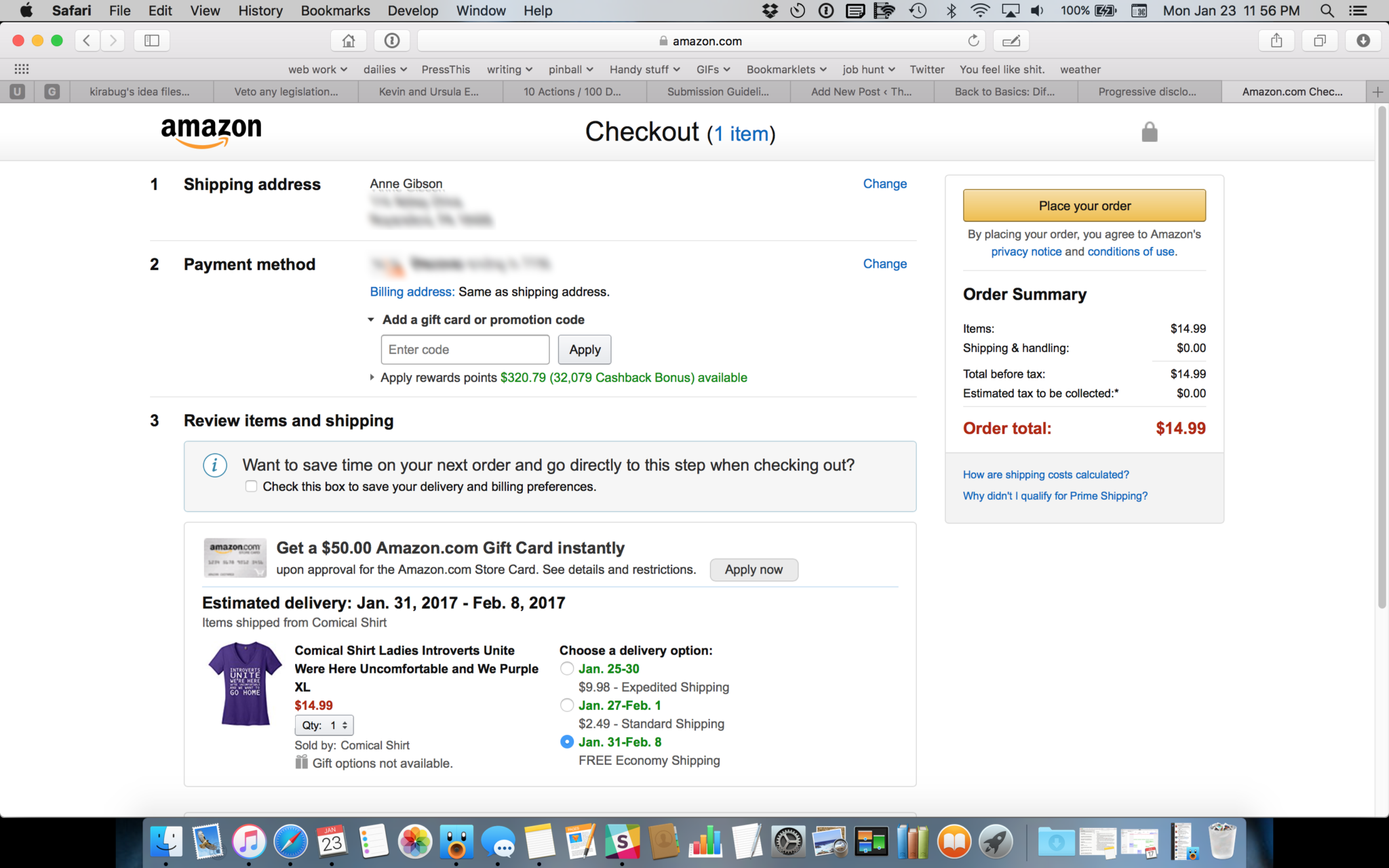This screenshot captures the checkout page on Amazon. Prominently displayed in the top left corner is the recognizable Amazon logo, featuring black text and the signature orange arrow curving in a U-shape. This page is identified as the checkout page, evident from the bold "Checkout" text situated at the top center. The user, Anna Gibson, appears to be purchasing a single item.

The shipping address section is blurred for privacy, revealing only Anna's name. Similarly, the payment method details are obscured. Under the payment method section, the billing address is indicated to be the same as the shipping address. There is an option available to add a gift card or promotional code, but it has not been utilized by the buyer.

Further down, in the "Review Items and Shipping" section, a gray notification box hints at a time-saving feature for future orders, suggesting the buyer check a box to save delivery and billing preferences for a quicker checkout process. This feature is often associated with Amazon’s "Buy Now" button, which enables a swift, almost one-click purchasing experience that bypasses several steps.

The item being purchased is described as a "Comical Shirt" for ladies, with the slogan "Introverts, Unite! We're Here, Uncomfortable, and We Purple." The shirt is in XL size and is shown in a purple color, adding a touch of humor and personality to the purchase.